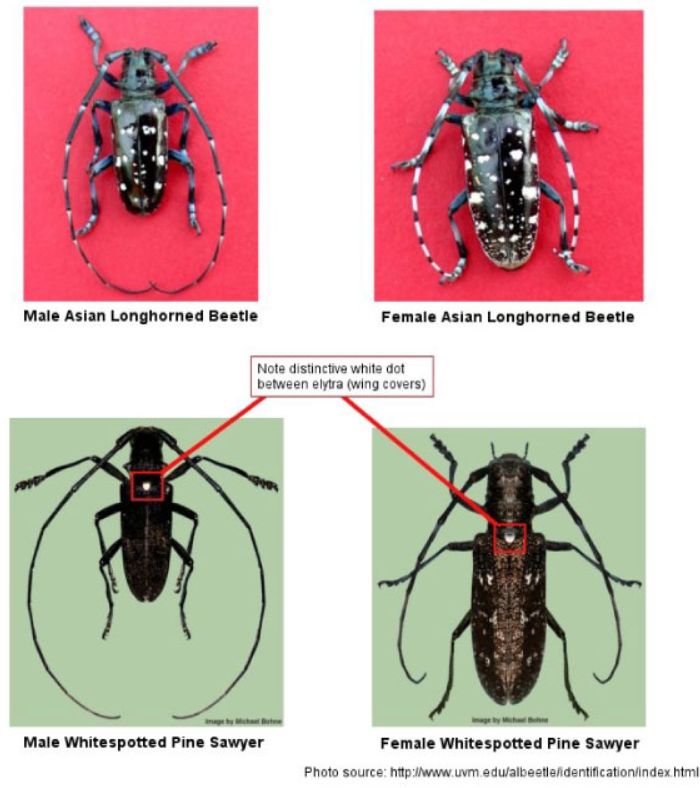This image is a compilation of four distinct photographs intended to identify different beetle species. In the top left corner, set against a red rectangle, is a black beetle with white spots and antennae longer than its body. This beetle is labeled "male Asian long-horned beetle" in a black caption beneath it. To the right, in the top right corner, is a similar beetle, also black with white spots, but with antennae as long as its body; it is captioned "female Asian long-horned beetle." In the bottom left corner, within a green rectangle, is a black beetle featuring a single white dot on its neck and long antennae, identified as the "male white-spotted pine sawyer." Lastly, the bottom right corner shows a larger beetle of the same species, labeled "female white-spotted pine sawyer."